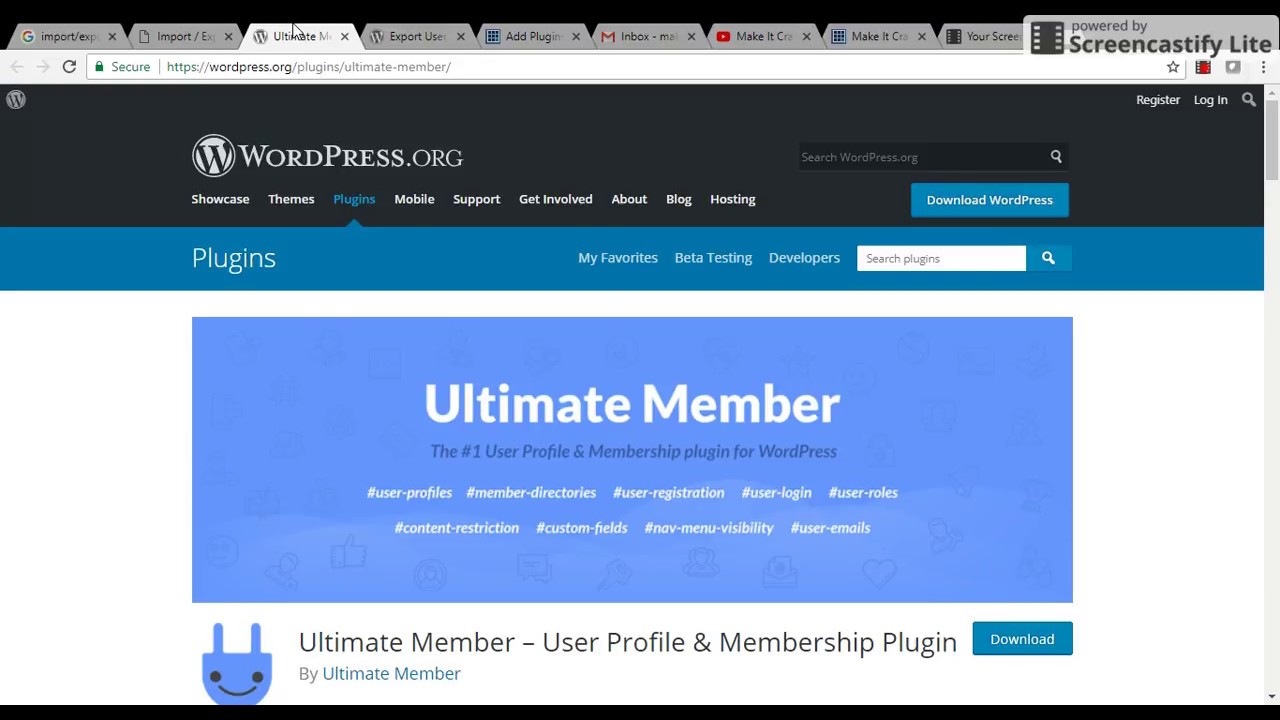This image is a screenshot of the WordPress.org website, specifically featuring the Ultimate Member plugin. Ultimate Member is highlighted as the top user profile and membership plugin for WordPress. The screenshot prominently displays the plugin's key features such as User Profiles, Member Directories, User Registration, User Login, and User Roles, each indicated by hashtags. Also visible is a dark blue box containing a download option for the plugin, allowing users to easily access and install Ultimate Member.